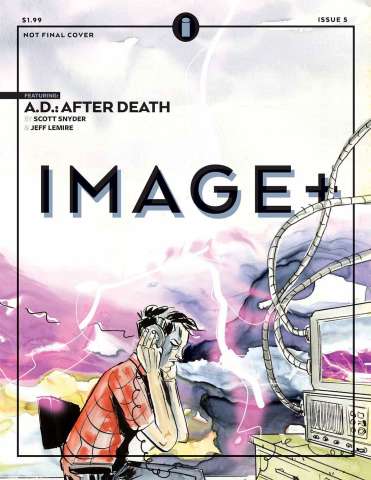The cover image is a meticulously hand-drawn illustration, framed by a thin black border. At the top of the image, black text prominently displays the following: "$1.99," "not final cover," "Issue 5," "A.D. After Death," "Scott Snyder," "Jeff Lemire," and "Image Plus." Centrally featured in the artwork is a watercolor depiction of a man wearing retro-style headphones, pressing them firmly onto his head. He is seated in a black office chair with armrests, intently facing a white, vintage computer adorned with thick, numerous cords originating from both the computer and a receiver-like device beneath the monitor. The desk holding the computer is light brown and positioned at the bottom of the illustration. The scene is accentuated with a vivid palette of black, gray, pink, purple, orange, and green. An additional detail includes a lowercase 'i' within a gray circle, situated at the top center of the cover, enhancing its distinct comic book style.